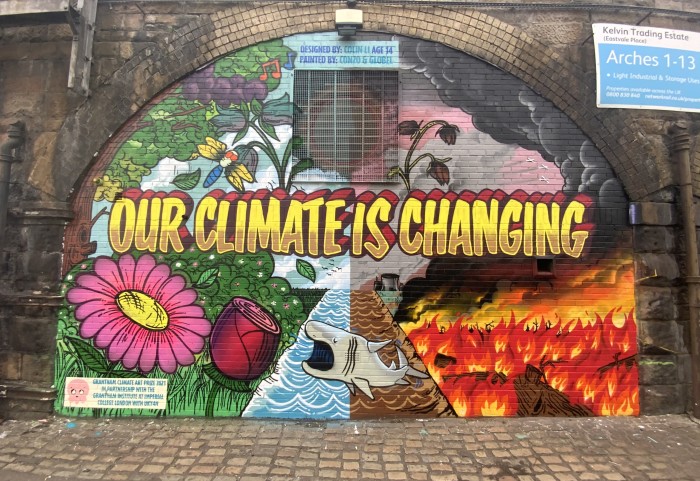The image captures a vibrant mural painted on the side of an old brick and stone building. The mural, which prominently features the text "Our Climate is Changing" in yellow and red, spans the space within an arch that formerly housed a window or doorway, now filled with bricks. Above the mural's arch, a sign reads "Kelvin Trading Estate, Eastvale Place, Arches 1-13, Light Industrial and Storage Units". Below the arch, another sign credits the mural's creation to "Design by Colin, age 14, painted by Colin and Gloria."

The mural itself is a poignant depiction of contrasting environmental scenes. On the right side, it portrays a grim, dystopian landscape with wildfires, barren plants, and dark smoke clouds, symbolizing environmental degradation. On the left, the scene transitions to a more hopeful and lush environment filled with greenery, flowering plants, fruit-bearing trees, and dragonflies, representing a thriving, healthy ecosystem. The lower part of the mural blends with these elements, showing water and a striking image of a whale. The foreground of the building is covered in a cobblestone pathway, adding to the rustic texture of the old building's exterior.